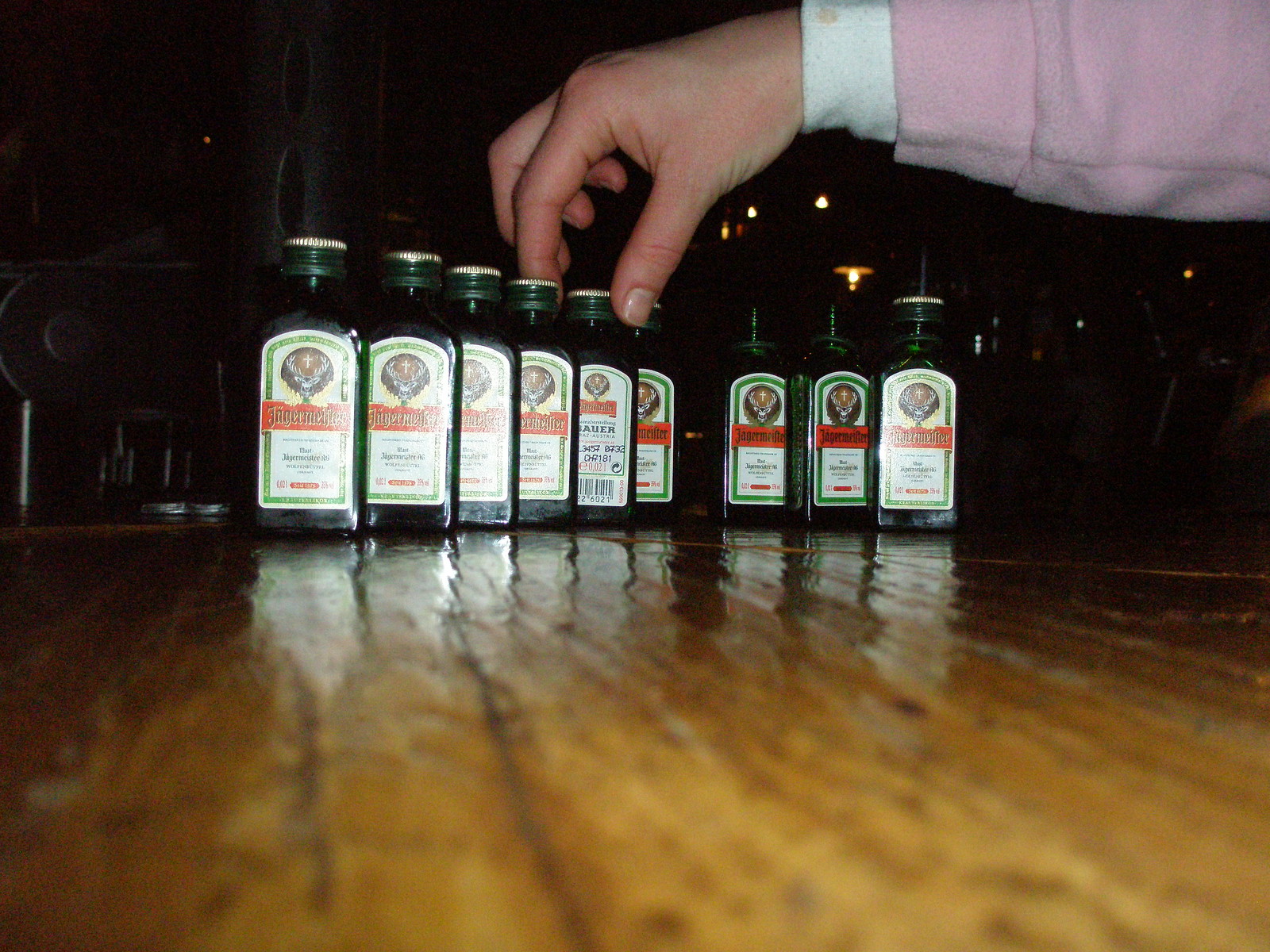This photograph captures a moment of preparation involving miniature bottles of Jägermeister, each characterized by their iconic dark green glass, adorned with a silver screw-on cap. The label on each bottle is distinctively red, featuring the brand name and a logo depicting deer antlers with a cross at the top. The setting appears to be the polished wooden surface of a bar counter, reflecting the bottles’ rich hues. In the foreground, an arm, clad in a soft, pinkish jacket with a white cuff peeking out from the sleeve, is seen meticulously arranging the bottle caps. The figure's gender is ambiguous. The background is predominantly dark, save for some muted gray shades and faint outlines of a room illuminated by ceiling lights on the right side of the image.